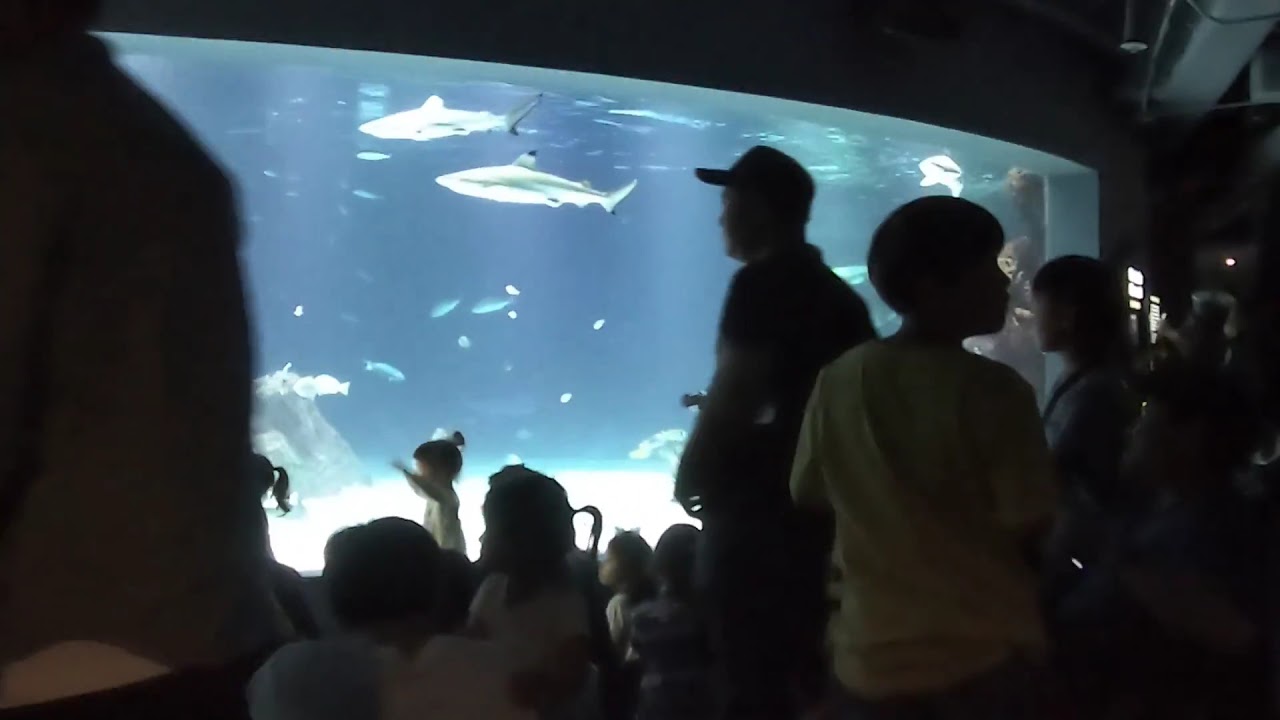In this photograph of an indoor aquarium, a crowd of people, including adults and children, are gathered and gazing intently at a large, brightly-lit tank that spans an entire wall. The vivid blue water and white sandy bottom of the aquarium are illuminated, serving as the primary light source in the otherwise dim room. Prominently visible in the center of the tank are two small gray and white sharks, with various other fish swimming below them; some are little blue fish, while others are more white in color, suggesting different species. 

The tank features a gray rock outcrop on the left side and a slightly curved shape, adding depth to the display. On the right side of the image, outside the tank, there is a door with a red light above it and a backlit information placard to its left. Among the observers, an adult wearing a baseball cap stands out as the tallest figure, while a child in a yellow short-sleeved t-shirt turns away from the tank, looking to the right. Closer to the aquarium, two young girls with ponytails are engrossed in the view, pressed up against the glass. The photo also captures the unfinished ceiling with visible air conditioning ducts and conduits, adding an industrial element to the setting. Through the crowd, we glimpse the vibrant underwater scene, creating a captivating contrast with the dark, out-of-focus figures in the foreground.